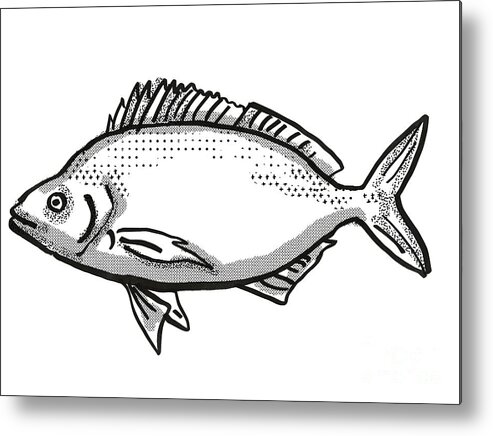This detailed black and white illustration of a fish occupies approximately 70% of the image, with the fish swimming towards the left. Its body is fuller and exhibits a slight smile, creating a sense of personality. The fish is illustrated on a white rectangular background and appears as if it could be computer-generated due to the uniform gray shading on its belly and fins.

The fish features a prominent eye, characterized by a black circle containing a white area and a central black dot, giving it a distinctive look. The fins on its back, resembling a dorsal fin, are shaded and extend along its top side, while a large, partially shaded v-shaped tail completes the fish's outline. Additionally, smaller fins are visible on the bottom and toward the lower back of the body.

Pixel-like dots across the upper part of the body add texture and depth, enhancing the detailed appearance of the fish. The overall effect of this illustration, with its sharp fins and meticulous shading, creates a visually engaging depiction of a seemingly "fat" fish from a side profile angle.